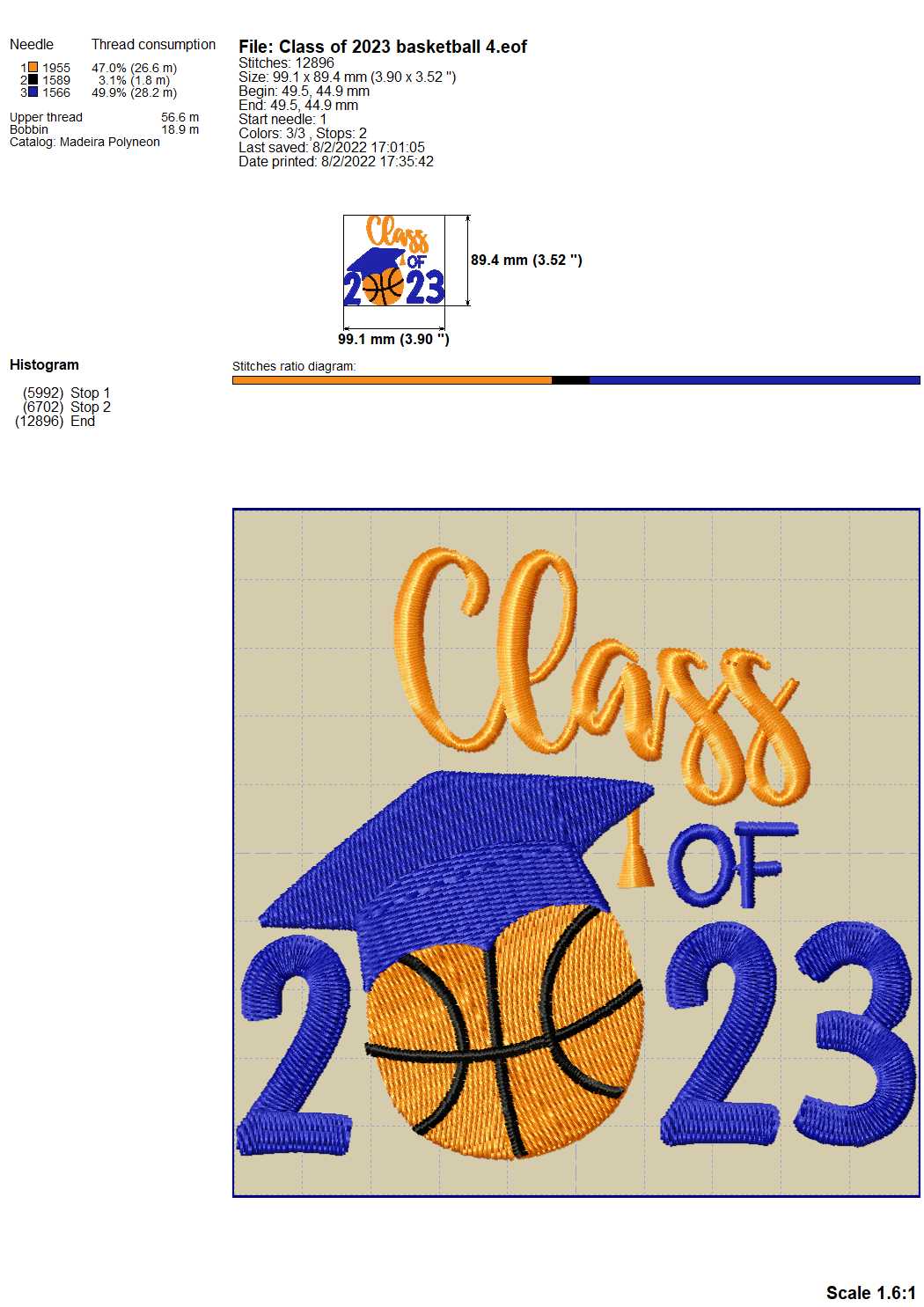The image features an intricately embroidered design with a yellowish-brown, square-patterned background. At the center, the text "Class of 2023" is prominently displayed, with "Class" in bright yellow cursive and "of 2023" in dark blue. The zero in "2023" is creatively depicted as an orange basketball wearing a dark blue graduation cap. Surrounding this playful yet elegant central motif is a detailed embroidery patch, showcasing the meticulous needlework. Above the main design, there's an overlay of technical specifications including the file name "classof2023basketball4.eof," along with details on stitches, thread colors, and needle usage. It lists statistics such as orange thread (26.6 meters, 47.0%), black thread (1.8 meters, 3.1%), and specifics like total size, stitch count, needle starts, and thread consumption. The overall composition presents a harmonious blend of creative design and precise technical embroidery details.